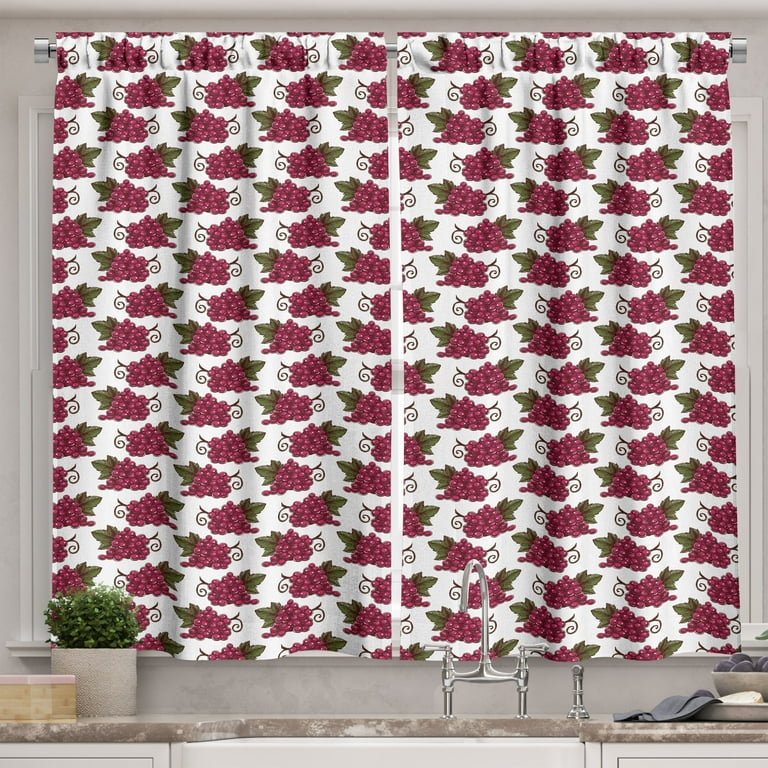The image depicts a kitchen scene centered around a window with white curtains decorated with a repeating pattern of purple grape clusters and green leaves, some facing left and some facing right. The window curtains are held by a metallic bar at the top. Below the window is a kitchen countertop made of gray and white marble, housing a silver faucet with a hook-like spout and a separate sprayer for washing dishes. On the lower left side of the counter stands a white pot containing a small flowering plant, while on the right side, there are trays with a grayish-blue matte cloth and a bowl filled with purple plums. Beneath the countertop are white cabinets. This detailed scene captures both functional and decorative elements of a neatly arranged kitchen space.